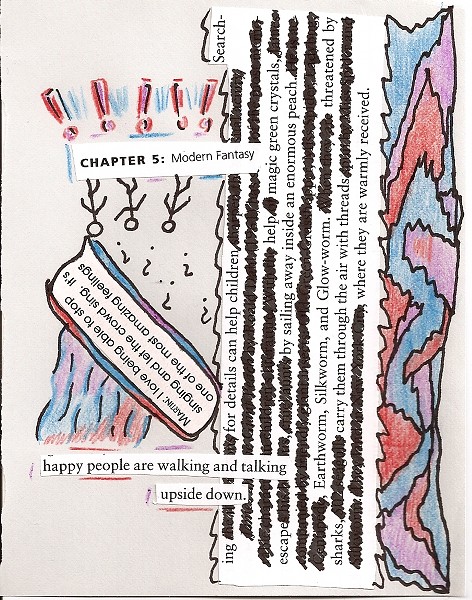The image is a mixed media collage titled "Chapter 5: Modern Fantasy" set against a white paper background. The upper left quadrant features hand-drawn exclamation points in red with blue shading. Below these, a cut-out typed label reading "Chapter 5: Modern Fantasy" appears to be either torn or carefully arranged. Beneath this label are three upside-down stick figures accompanied by upside-down question marks. The leftmost stick figure has a voice bubble framed in crayon-like red, blue, and purple, which reads, "Martin: I love being able to stop singing and let the crowd sing. It's one of the most amazing feelings." Directly below this bubble is a rainbow-colored waterfall depicted in purple, blue, and red hues. Under the waterfall, another piece of cut-out text states, "happy people are walking and talking upside down."

The entire right section of the artwork is divided into two vertical strips. The central strip contains redacted, hand-fashioned typed words, with certain phrases remaining legible: "Searching for details can help children, help magic green crystals escape by sailing away inside an enormous peach, earthworm, silkworm, and glowworm threatened by sharks carry them through the air with threads where they are warmly received." Adjacent to this text, the rightmost strip showcases jagged hand-drawn lines shaded in colors matching the previously used purples, blues, and reds. The left section of the background is predominantly pink, contrasting against the vivid colors and eclectic textual elements that create an abstract and whimsical composition.